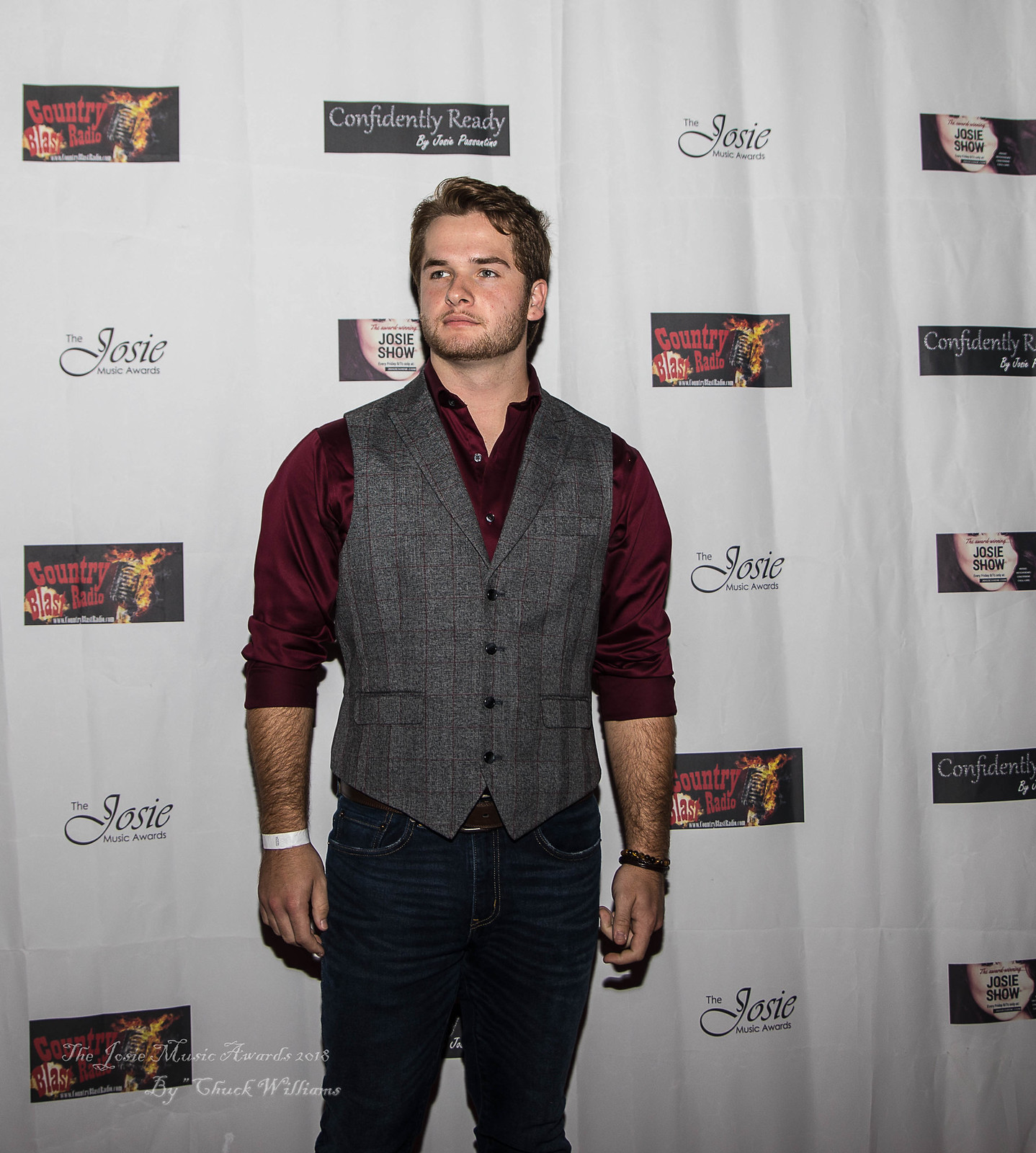In this image, a man is standing slightly off-center to the left, facing the camera. He has short brown hair and some facial hair. The man is dressed in a gray vest with black accents and pockets, over a maroon undershirt, and dark blue jeans. He is accessorized with a white wristband on his right arm and beads on his left hand.

The background is a large, white banner featuring various elements of promotional text. At the top left of the banner, the words "Country Blast Radio" are prominently displayed in red, black, and orange. To the top right, adjacent to the "Josie Show" logo, is the "Josie Music Awards." Above the man's head, the banner reads "Confidently Ready by Josie Passantino." Additionally, in the bottom left corner, the text "The Josie Music Awards 2018 by Chuck Williams" is visible. This setting suggests that the man is posing at a country music awards event.